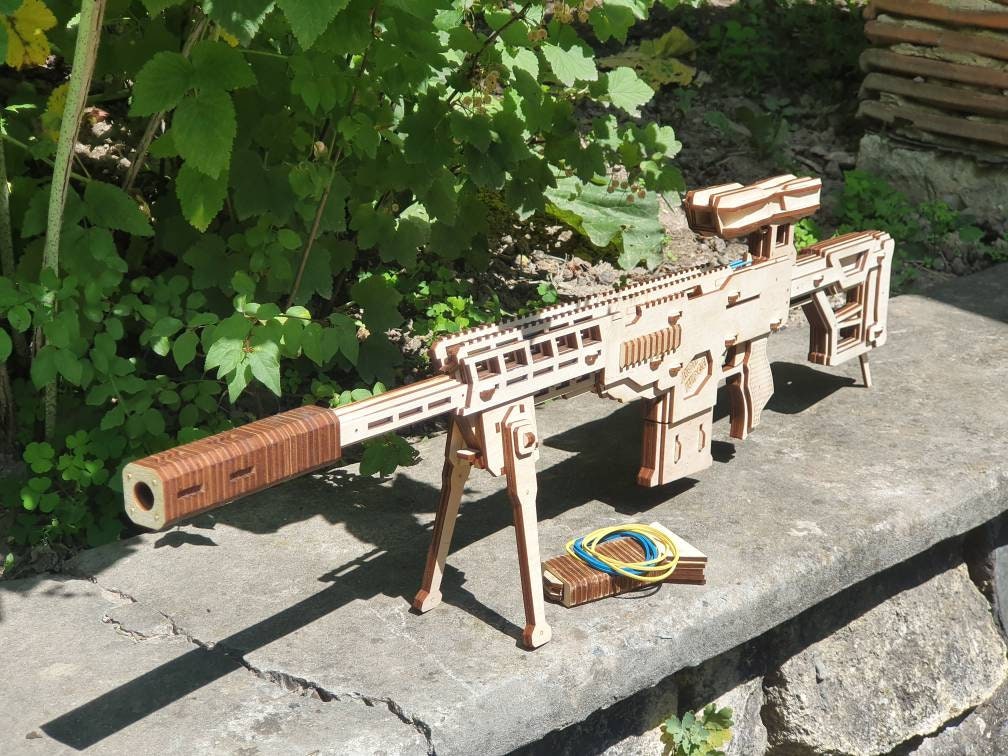This is an outdoor photographic image featuring a meticulously crafted replica of a machine gun. The gun, primarily light beige in color with a dark brown silencer-like tip at the end of its notably long barrel, is designed to resemble a potentially non-functional weapon that might be made from wood. The end of the barrel appears thicker and is distinguished by the brown color. The gun is mounted on a stone wall, supported by two front legs under the barrel and a single back leg under the gun stock, giving it stability. A magazine is visibly located in the center of the gun, which appears to be pointing diagonally from the top right towards the middle bottom left of the image. Resting on the gray stone surface beneath the gun are brown cards, possibly suggesting bullets, and a yellow and blue band of wires that resemble rubber bands, hinting that the gun might shoot rubber bands. In the background, a stone wall and a tree with blue-green leaves are visible, alongside a small wooden structure. The scene evokes a historical aesthetic, perhaps suggestive of World War II, set against an outdoor backdrop with no added text.